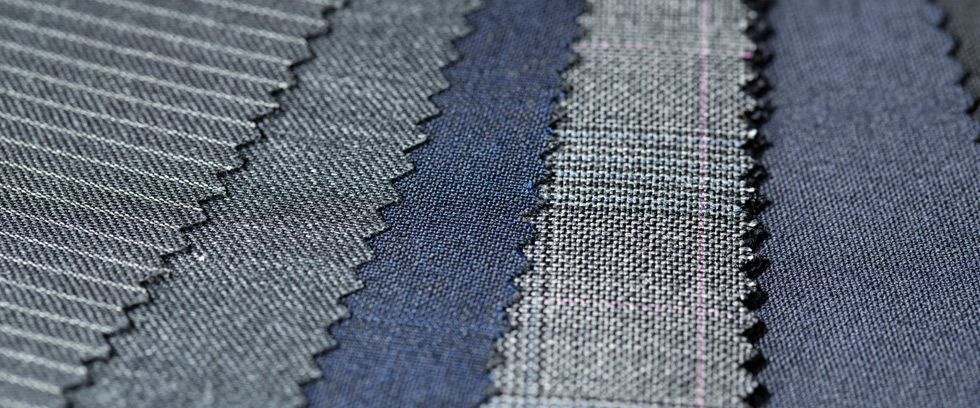This photograph showcases five overlapping pieces of fabric, each with distinct colors and patterns, filling the entire image except for the very upper right corner which is a plain dark gray. The fabrics are cut with pinking shears, giving them a notched edge. Starting from the right, the first fabric is a blue denim. Next to it, overlapping to the left, is a faint black and white plaid fabric with a light pink vertical stripe. Continuing leftward, there is a darker blue denim piece. Moving further left, there's a black and white fabric with a salt-and-pepper appearance. Lastly, occupying the upper left corner and extending down to the bottom left is a dark gray fabric adorned with thin horizontal white stripes.